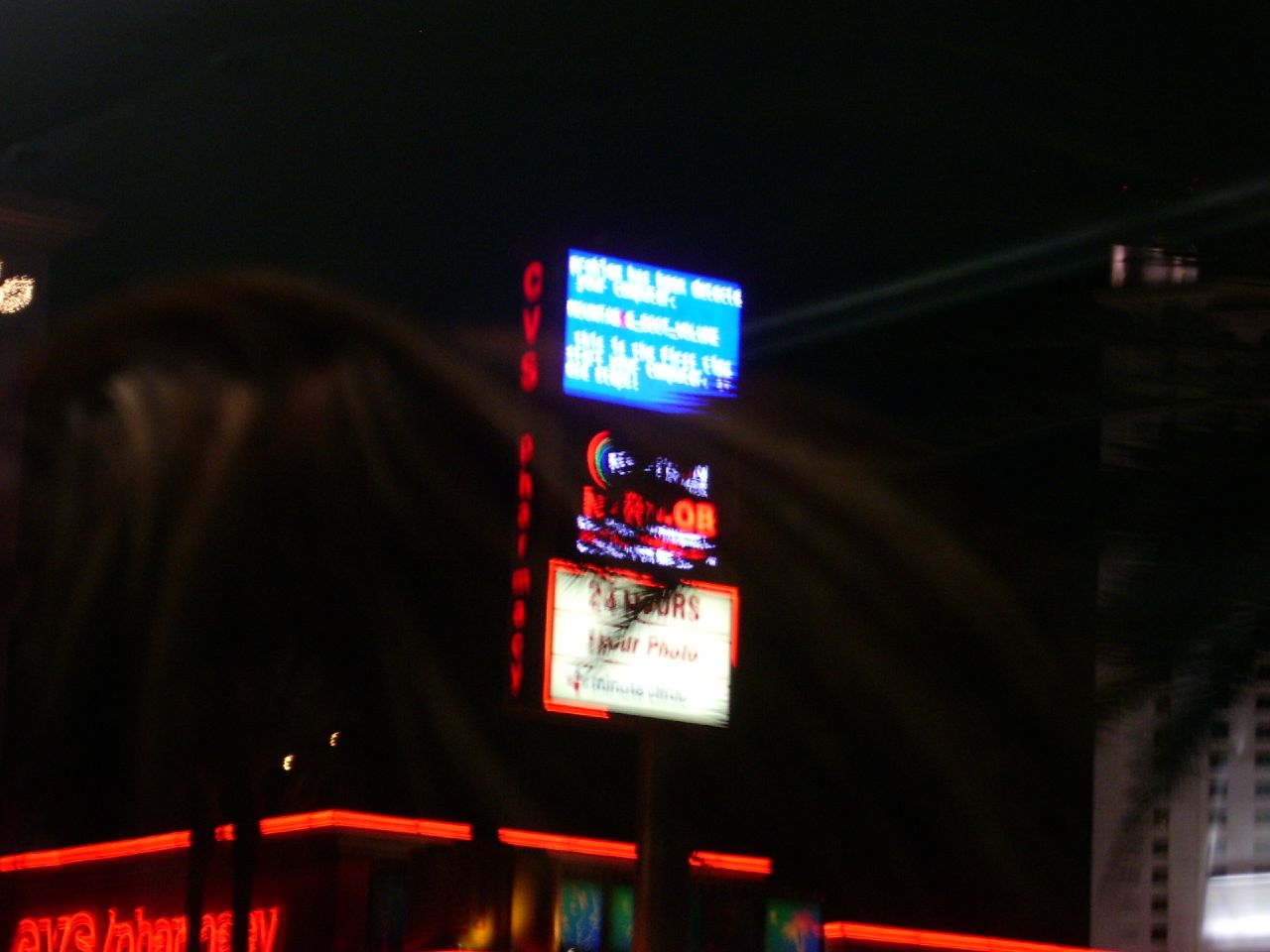This photograph, taken at night, captures an outdoor view with a jet-black sky as the backdrop. The central focus is a three-tiered sign outside a business, partially obscured by the curled, brown leaves of a nearby palm tree. Additional foliage on the right side of the image somewhat masks a tall, gray building that remains indistinct. At the bottom of the image, there's a building adorned with bright red LED lights outlining its roof, accompanied by a red LED sign with partially cut-off lettering. The top tier of the sign prominently displays "CVS Pharmacy" in red, along with "24-hour photos." A blue screen with white, unreadable print is also visible on the sign, adding to the nighttime ambiance.